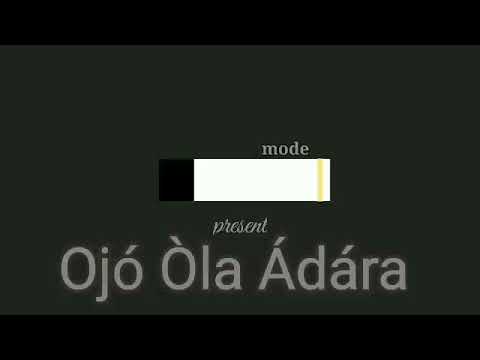The image appears to be a sign featuring a color adjustment slide. The background is dark gray with black bars at the top and bottom. Dominating the image is a large gray rectangle. At the center of this rectangle, there's a horizontal bar that transitions from pitch black on the left to white across most of its length, ending with a narrow vertical yellow stripe on the far right. Above this bar, in light gray lowercase letters, is the word "mode." Below the bar, written in a flowing script, is the word "present." Underneath that, in another language, are the words "Ojó, Olá, Ádara," with accent marks on the second 'O' in "Ojó," the first 'O' in "Olá," and the leading 'A's in "Ádara."